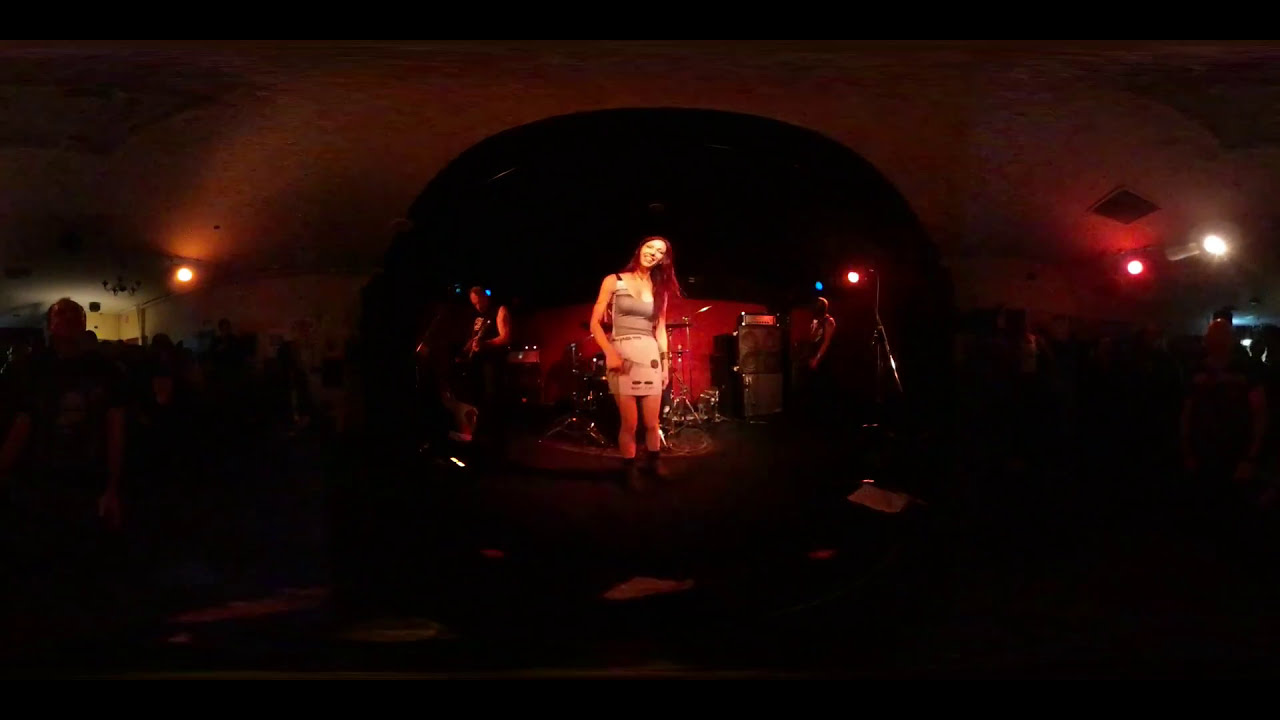The image is a photorealistic capture of a dark indoor club featuring a musical performance on a circular center stage. The stage is moderately well-lit with red and white lights on the right, and orange and yellow lights on the left, casting a dramatic ambiance. Dominating the center stage is a young woman with long red hair, dressed in a gray tank top and a white skirt, smiling and slightly inclining her head to the right. She appears to be the lead singer, possibly holding a microphone, and seems aware of the camera, posing gracefully. Behind her, a partially visible man in a dark shirt is playing the guitar. A drum set is positioned immediately behind her, though it's largely obscured by her presence. On the stage's right corner, another man stands next to some speakers, partially hidden in the shadow. The backdrop of the stage is red, contrasting the overall dim, black surroundings which obscure the audience. A significant dark semicircle, likely the roof of the club, arches above, completing the moody, intimate setting of the performance.